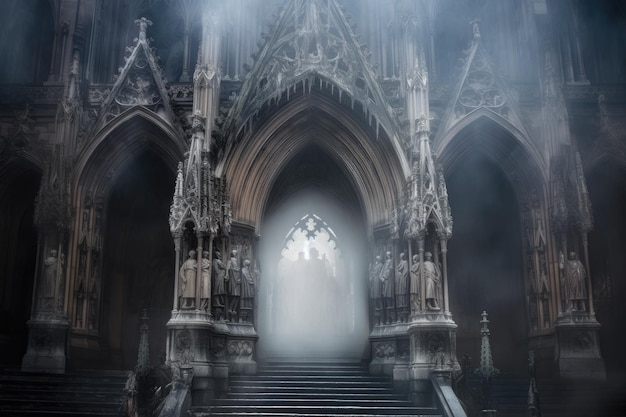This horizontal rectangular image depicts the facade of a Gothic cathedral, characterized by its intricate medieval architecture. At the heart of the scene, three pointed archways create a dramatic entryway, with the central archway being notably larger and flanked by two smaller ones. A series of steps lead up to this central arch, which is enveloped in a mysterious white haze or smoke, adding an ethereal quality to the atmosphere. The presence of a hazy, indistinct figure in white robes can be faintly discerned through the mist, standing inside the bright-lit central archway.

On either side of the central archway, the two smaller arches are shrouded in darkness, accentuating the stark contrast between them and the illuminated center. Elegantly carved statues adorn the sides of these archways, particularly around the central entrance, where at least ten statues are embedded into the inner walls. The facade itself combines dull hues of brown, black, beige, and gray, contributing to the overall dark and moody tone of the image.

The detailed carvings and statues, along with pointed, intricate designs such as triangles, enhance the grandeur of the cathedral's architecture. The ambiguity of the perspective—whether the viewer is inside looking out or outside looking in—adds an intriguing, mysterious element to the scene, consistent with the European medieval design ethos.